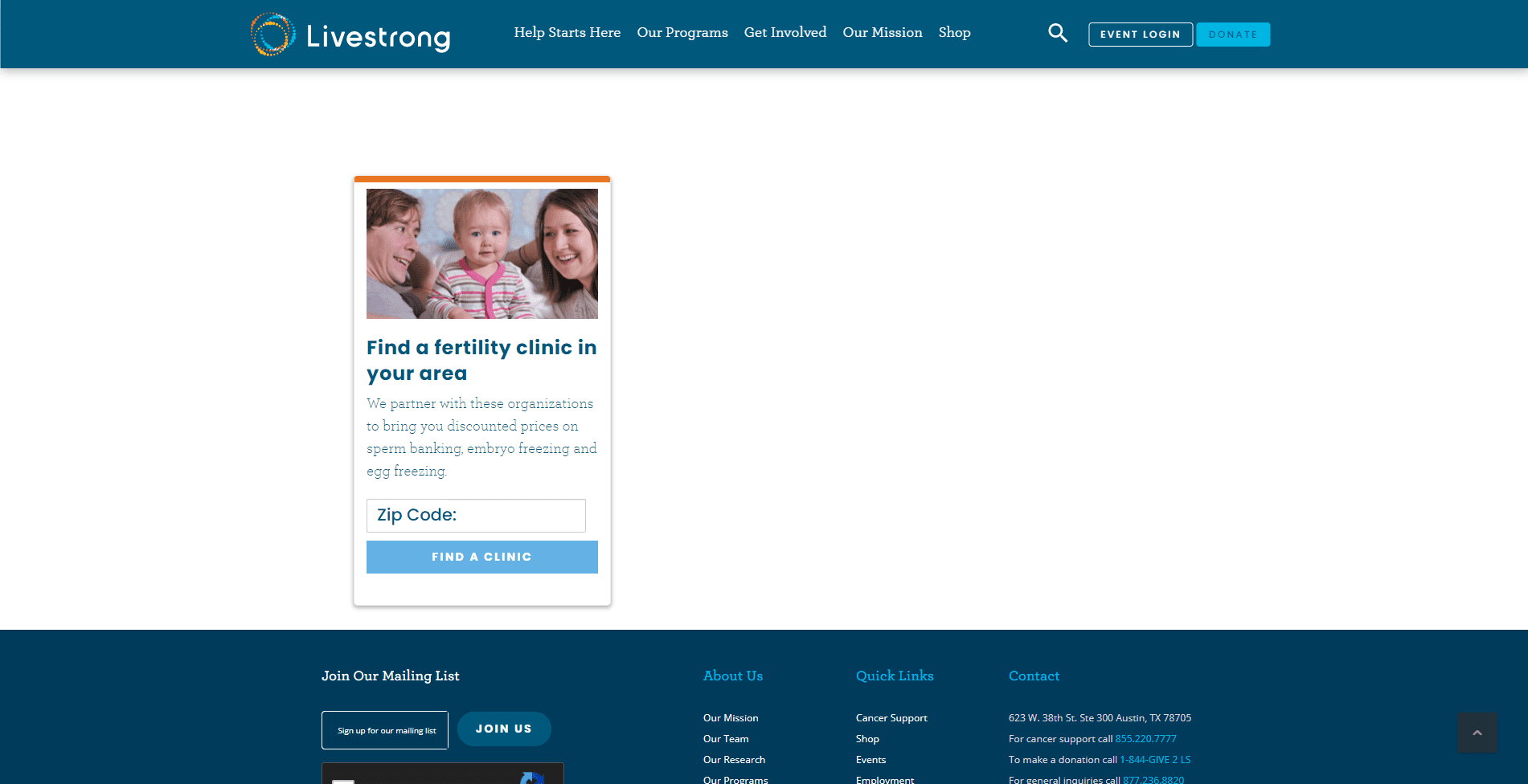The image showcases a medical-themed website for Livestrong. The top navigation bar is a greenish-blue hue, with the Livestrong logo positioned at the top left in white text. Adjacent to the logo is an emblem consisting of an orange circle faintly overlaid on a blue circle, with a very faint reddish-orange circle at the center, and the lines of the design are not solid.

The main menu features options including "Help Starts Here," "Our Programs," "Get Involved," "Our Mission," and "Shop." Additional options on the same bar include "Login," "Donate," and an event section. The central background of the main screen is white, highlighting a singular post.

At the top of the post is an orange strip, followed by a photograph depicting a family: a mother, a father, and a very young child with blonde hair, appearing to be around two years old or possibly younger. The post title reads, "Find a Fertility Clinic in Your Area." The accompanying text explains that Livestrong partners with various organizations to offer discounted prices on sperm banking, embryo freezing, and egg freezing. Below the text, users can input their zip code to locate a nearby clinic.